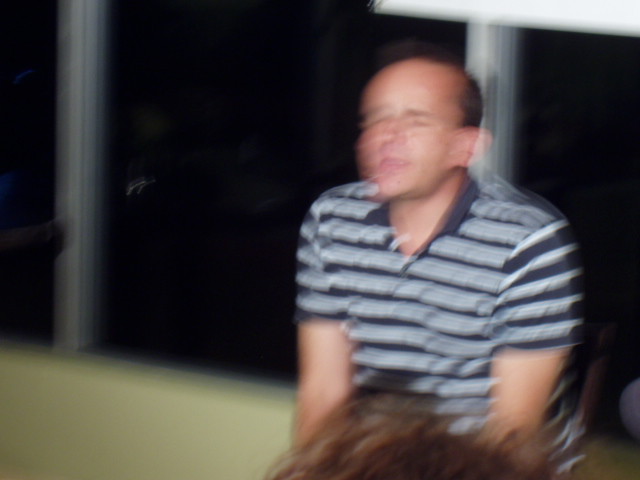The image depicts a blurry photograph likely taken with a moving camera, rendering the image’s quality quite poor. Despite the blur, the subject is identifiable: a bald, white man with sparse hair behind his ears and none on the top of his head. His facial expression conveys joy or amusement, as indicated by his closed eyes and open mouth, seemingly caught mid-laugh. He is dressed in a t-shirt featuring a dark blue collar and grey and blue stripes. The background shows a window with three glass panes, but the view outside is obscured by darkness. In front of the man, there is a yellow panel and an indistinct mass of hair. This hair could belong to another person, an animal, or possibly be a wig he is interacting with. Overall, the scene captures a candid moment filled with motion and obscured details.